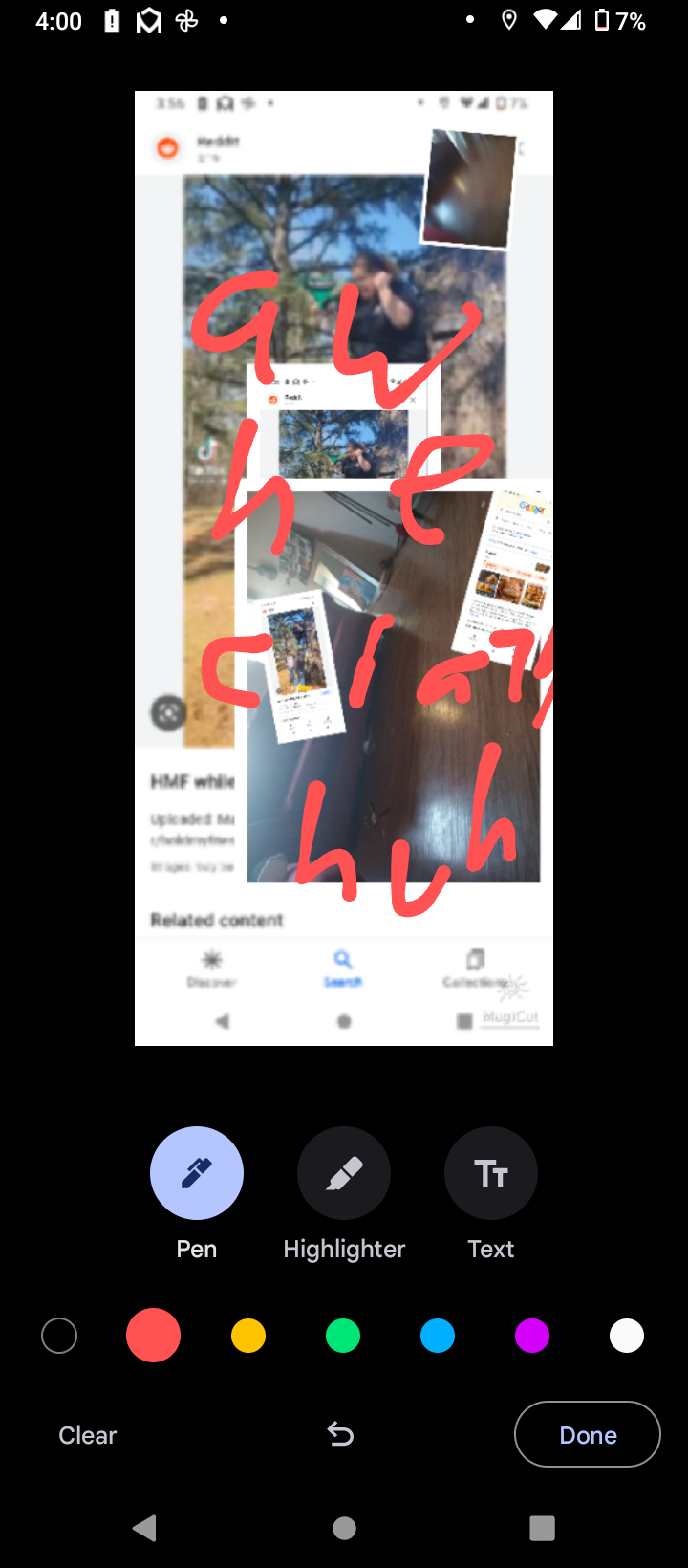The image showcases a phone screen displaying a photo editing interface. At the very top of the screen, typical cell phone icons are visible, indicating a time of 4:00 PM in the top left corner. To the right of the time, there are several white icons, followed by a Wi-Fi signal icon. The battery percentage, displayed at 7%, is located in the top right corner.

Beneath the status bar, there is a rectangular picture with red marker annotations that spell out "A-W-H-E-C-L-A-7" against a white background. Below the picture, a toolbar offers three editing options labeled "Pen," "Highlighter," and "Text," accompanied by six color choices in pink, yellow, green, blue, purple, and white circles.

Further down the interface, there are buttons labeled "Clear," a backward arrow symbolizing undo, and "Done." At the very bottom, navigation icons including a left arrow, a circle, and a square are set against a black background.